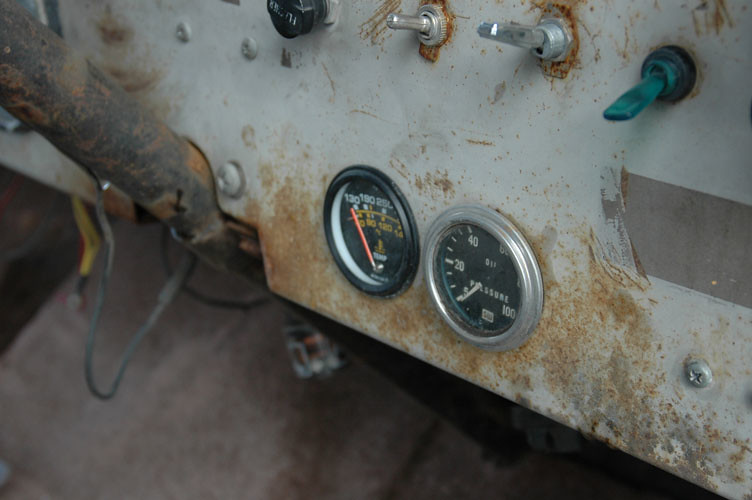The image showcases an aged and rusted control panel, likely from an old airplane or vehicle. A corroded pole, presumably the steering mechanism, prominently extends from the central area. To the right, there is a white metal dashboard, whose surface is heavily weathered and adorned with numerous screws. The dashboard is characterized by prominent rust, particularly at the bottom and around the switches.

At the top of the dashboard, a few silver switches are visible alongside a large green switch and a noticeable black button. Below these switches, there are two distinct gauges. The gauge on the left, which has a scale starting at 130 and reaching at least 250 (though the exact upper limit is not visible), is currently indicating a reading of 130. This measuring device is evidently used for temperature or pressure monitoring.

The gauge on the right is identified as a pressure gauge, with a scale ranging from 0 to 100. Its design features a silver outline with a black background and white text. This gauge is currently showing a pressure reading of zero.